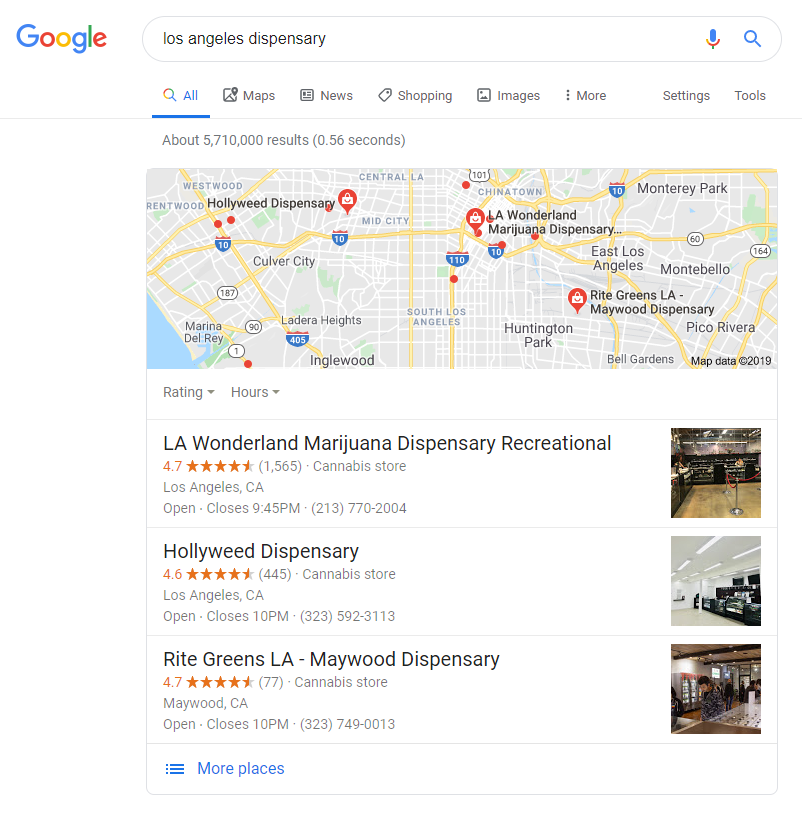This image appears to be a Google search results page for "Los Angeles dispensary." In the top left corner, the iconic Google logo is displayed with a capital blue 'G,' followed by lowercase letters in red, yellow, blue, green, and red respectively. The search query "Los Angeles dispensary" is entered in the search bar. The results indicate approximately 5,710,000 listings found in 0.56 seconds.

Featured prominently is a map pinpointing several dispensaries: Hollyweed Dispensary, LA Wonderland Marijuana Dispensary, and Wright Greens LA Maywood Dispensary. Each listing includes a dropdown arrow for ratings and hours of operation.

Detailed information about the dispensaries is provided:

1. **LA Wonderland Marijuana Dispensary**
   - **Rating:** 4.7 stars out of 1,565 reviews
   - **Description:** Cannabis store located in Los Angeles, California
   - **Hours:** Open until 9:45 PM
   - **Phone Number:** (213) 770-2004
   - **Image:** A photo of the establishment is displayed to the right

2. **Hollyweed Dispensary**
   - **Rating:** 4.6 stars out of 445 reviews
   - **Hours:** Open until 10:00 PM
   - **Phone Number:** (323) 592-3113
   - **Image:** A photo of the establishment is shown

3. **Wright Greens LA Maywood Dispensary**
   - **Rating:** 4.7 stars out of 77 reviews
   - **Location:** Maywood, California
   - **Hours:** Open until 10:00 PM
   - **Phone Number:** (323) 749-0013
   - **Image:** A photo of the establishment is provided

At the bottom left of the image, there is a blue hyperlink labeled "More places" which allows users to view additional dispensaries.